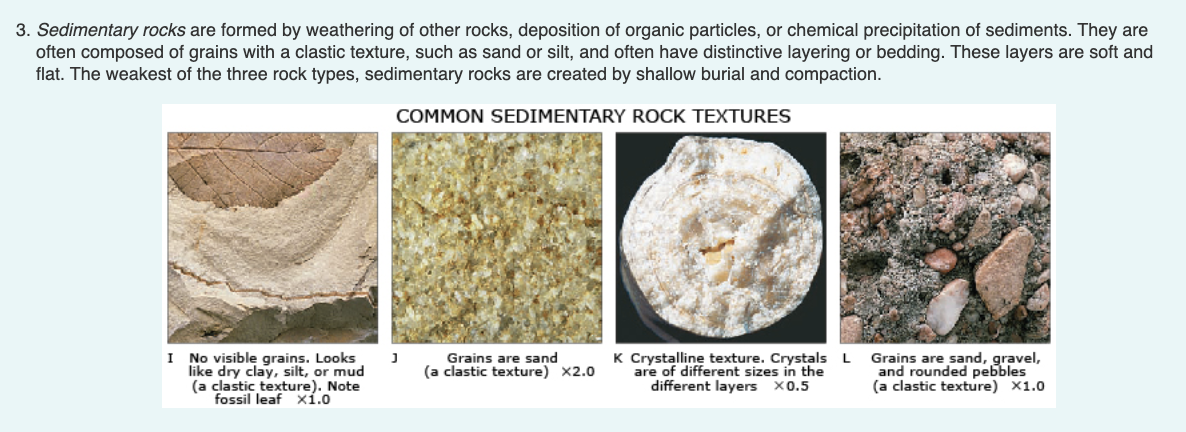The image displays a series of four side-by-side photographs showcasing different textures of sedimentary rocks, framed by a white border with the text "Common Sedimentary Rock Textures" in black font. At the top of the image, a caption explains that sedimentary rocks are formed by weathering, deposition of organic particles, or precipitation of sediments. These rocks are characterized by their grainy, classic textures such as sand or silt, distinctive layering, and they are the weakest and softest of the three rock types, often created by shallow burial and compaction.

The first photograph shows a rock with no visible grains, resembling dry clay, silt, or mud, with a classic texture and a fossil leaf, viewed at 1.0 magnification. The second photograph is a close-up of sand grains with a rough texture, magnified at 2.0. In the third photograph, a crystalline texture is depicted, where crystals of varying sizes can be seen against a black background, reminiscent of looking into a sushi roll filled only with rice, magnified at 0.5. The final photograph displays a mixture of sand, gravel, and rounded pebbles, presenting a classic texture at 1.0 magnification.